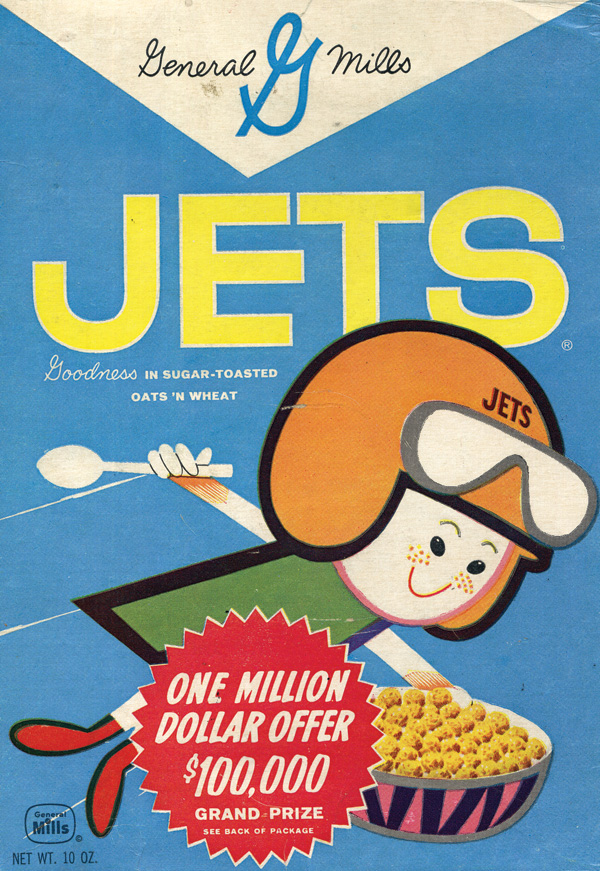This vintage advertisement, likely from the 1940s or 1950s, features Jets cereal by General Mills. The top of the poster showcases the distinctive General Mills logo, including an uppercase "G" in blue, set against a white, beigey triangle background. Below the logo, the word "Jets" stands out prominently in bright fluorescent yellow, bold, uppercase letters. Directly underneath, in white text, it reads, "goodness and sugar toasted oats and wheat."

The central image is a vibrant and playful depiction of a young boy in mid-flight, evoking a superhero aesthetic. He wears an orange helmet with "Jets" inscribed on it and matching goggles perched on top. The boy sports a green top, red shoes, and a wide, enthusiastic smile. Clutched in one hand is a navy blue and red-striped bowl filled with round cereal balls, while the other hand firmly grasps a spoon.

The composition is accentuated by a striking red starburst at the bottom announcing a "1 million dollar offer," with a $100,000 grand prize and a note to see the back of the package for details. The advertisement also lists the net weight as "10 ounces" in black text at the bottom left, beside another General Mills logo.

Overall, the ad combines dynamic imagery with bold, nostalgic colors and playful typography, capturing the essence of mid-20th-century marketing.